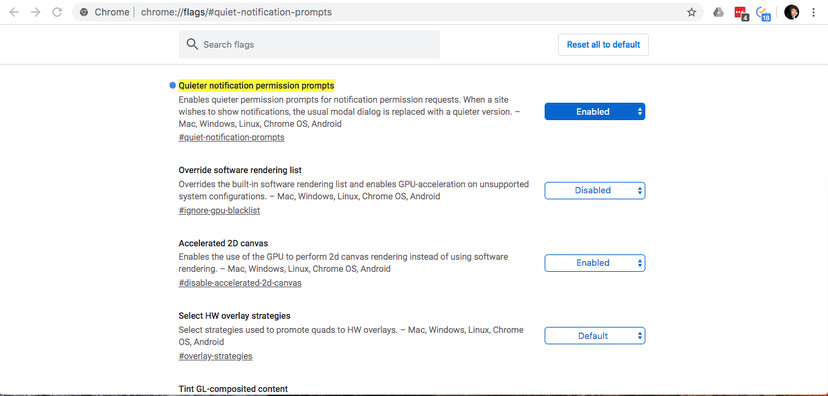In the image, we can see a section of Chrome's developer tools specifically dealing with feature flags and settings. The screenshot features the "Chrome Quiet Notification Prompt" section, allowing developers to fine-tune notification behaviors and rendering options. 

1. **Search Bar and Control Buttons**: At the top, there's a search bar enabling the search of specific feature flags. Adjacent to it is a "Reset all to default" button, which reverts any changes back to the original/default state.
   
2. **Quieter Notification Permission Prompts**: This feature is enabled and it simplifies the notification permission request process. When a site requests to show notifications, the typical modal dialog is replaced by a quieter, less intrusive prompt. This setting applies across multiple platforms: Mac, Windows, Linux, Chrome OS, and Android.

3. **Override Software Rendering List**: This disabled feature allows users to override the built-in software rendering list to enable GPU acceleration on unsupported system configurations. Like the quieter notifications feature, it is available on Mac, Windows, Linux, Chrome OS, and Android.

4. **Accelerated 2D Canvas**: Enabled by default, this feature leverages the GPU to perform 2D canvas rendering instead of relying on software rendering, enhancing performance. It is supported across Mac, Windows, Linux, Chrome OS, and Android.

5. **Select HW Overlay Strategies**: This setting, currently set to default, allows the selection of strategies used to promote quads to HW (hardware) overlays, optimizing the rendering process. It supports the same range of platforms: Mac, Windows, Linux, Chrome OS, and Android.

The detailed snapshot comprehensively captures the various developer options available for tweaking Chrome's behavior and performance preferences.